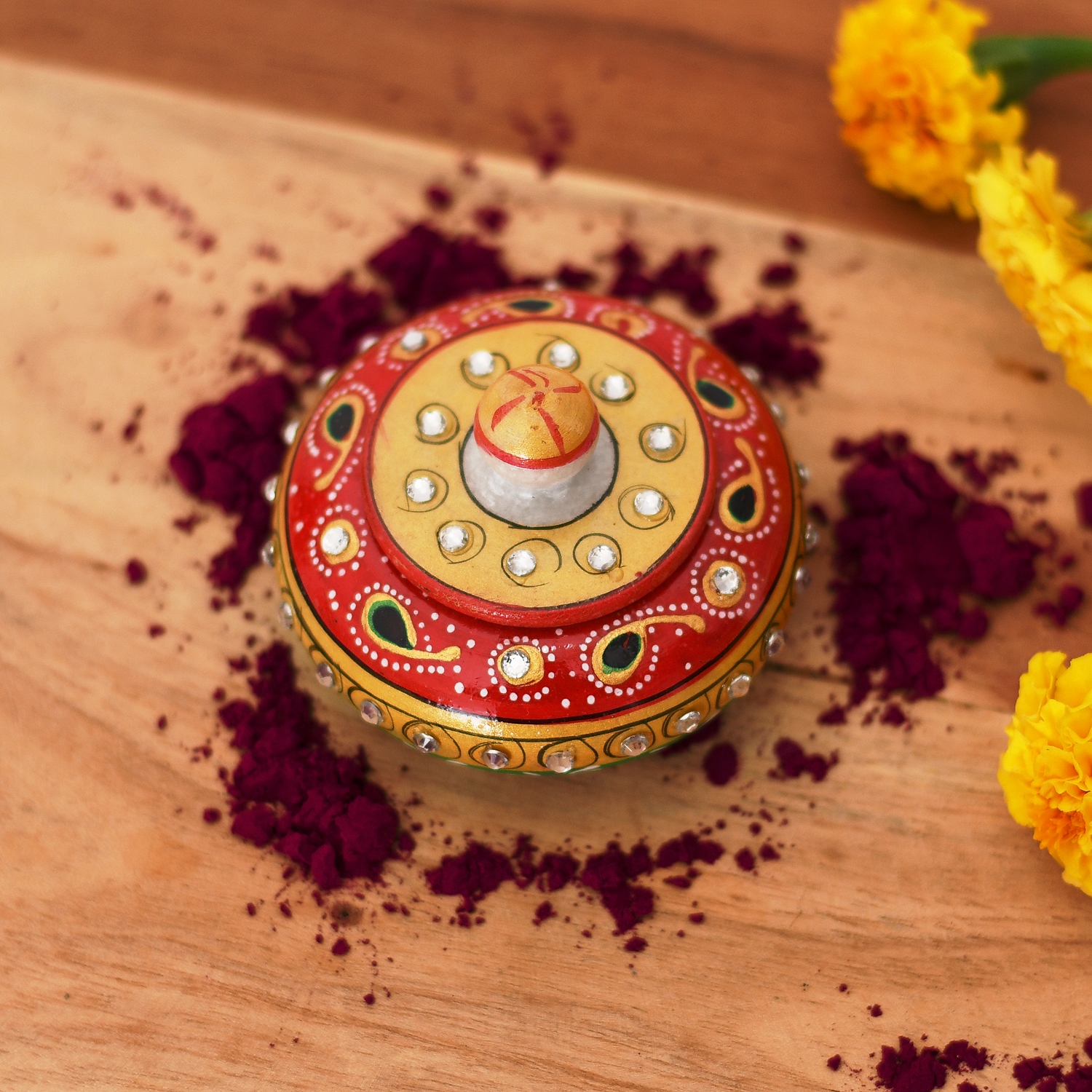In the center of the image is a small, round bowl intricately painted to resemble a sombrero. The bowl is made from light brown carved wood and features a closed, circular lid with a small, round handle on top. The lid's design is highly ornate, detailed with a central peak adorned with five red lines radiating outwards. This peak is surrounded by a white centerpiece with a black outline, encircled by ten black circles each containing a white gem. Encircling this white array is a yellow area dotted with white spots, followed by a red band with alternating embedded yellow gems, each with white dots. Tiny black and white ovals are also dispersed throughout this design, featuring white dots around them, contributing to an overall white, gold, and red stripe pattern. 

Surrounding the bowl is a fine brown powder, potentially coffee or dark brown sugar, resting on a flat wooden surface that exhibits a mix of light and dark wood grains. Adding a touch of vibrancy are three yellow flowers, one near the top right corner with its green stem slightly visible, and more flower tops peeking into the lower right area.

This vibrant, Hispanic-style bowl, possibly reminiscent of Mardi Gras decorations with its elaborate use of red, yellow, green, and black details, sits elegantly amidst its earthy and colorful surroundings on a diagonally dual-toned brown wooden background.